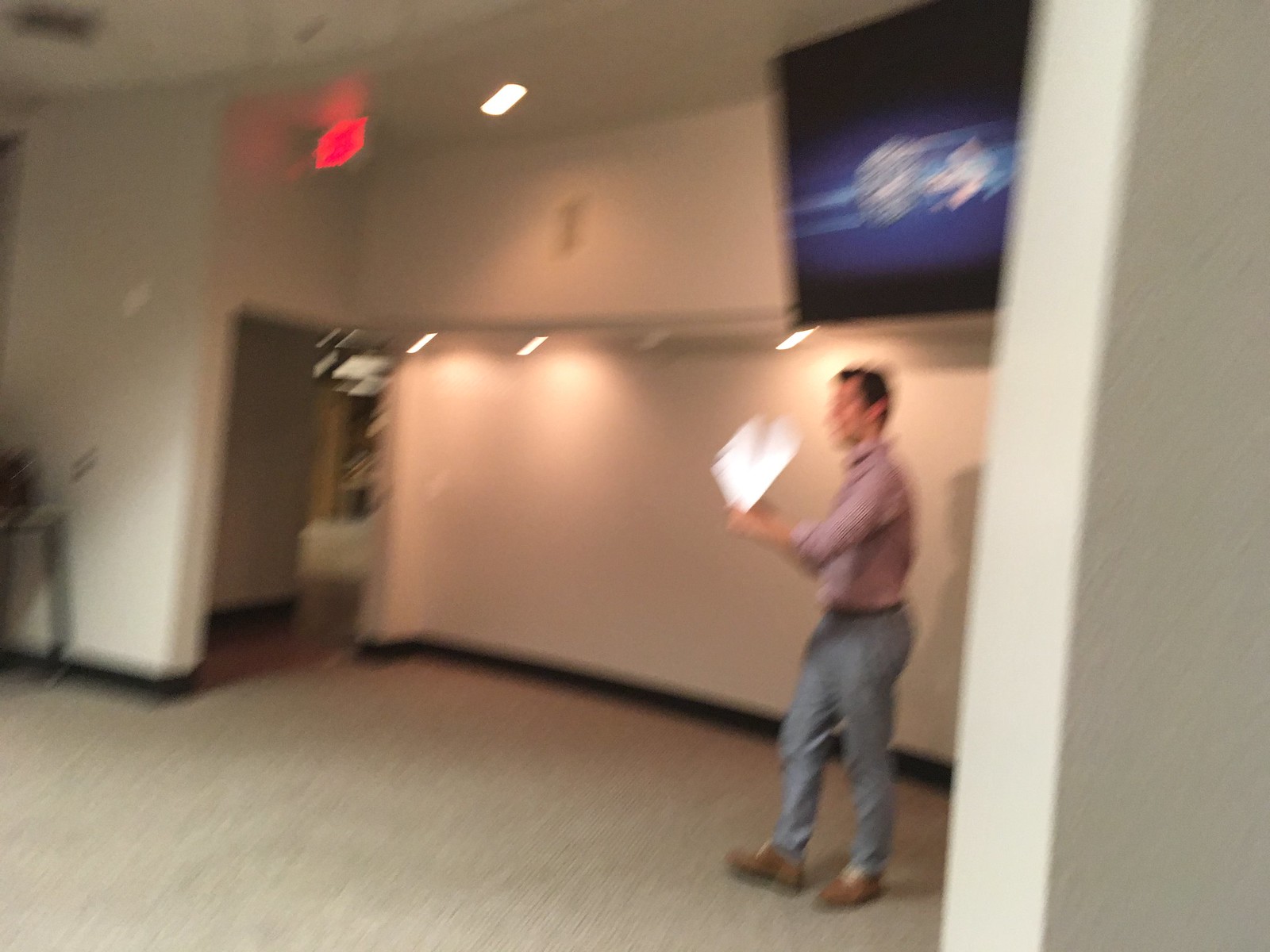This photograph is slightly out of focus, capturing a man standing in a hallway. The man is dressed in gray pants and brown shoes with white laces. He is wearing a long-sleeved reddish button-up shirt tucked into his pants. His hair is short and brown. Though the image is blurred, he appears to be holding a white piece of paper in his hand. The hallway features gray carpet flooring, black baseboards, and white walls. The hallway is well-lit, with an exit sign visible above. Across from the man, a doorway presumably leads to another room.